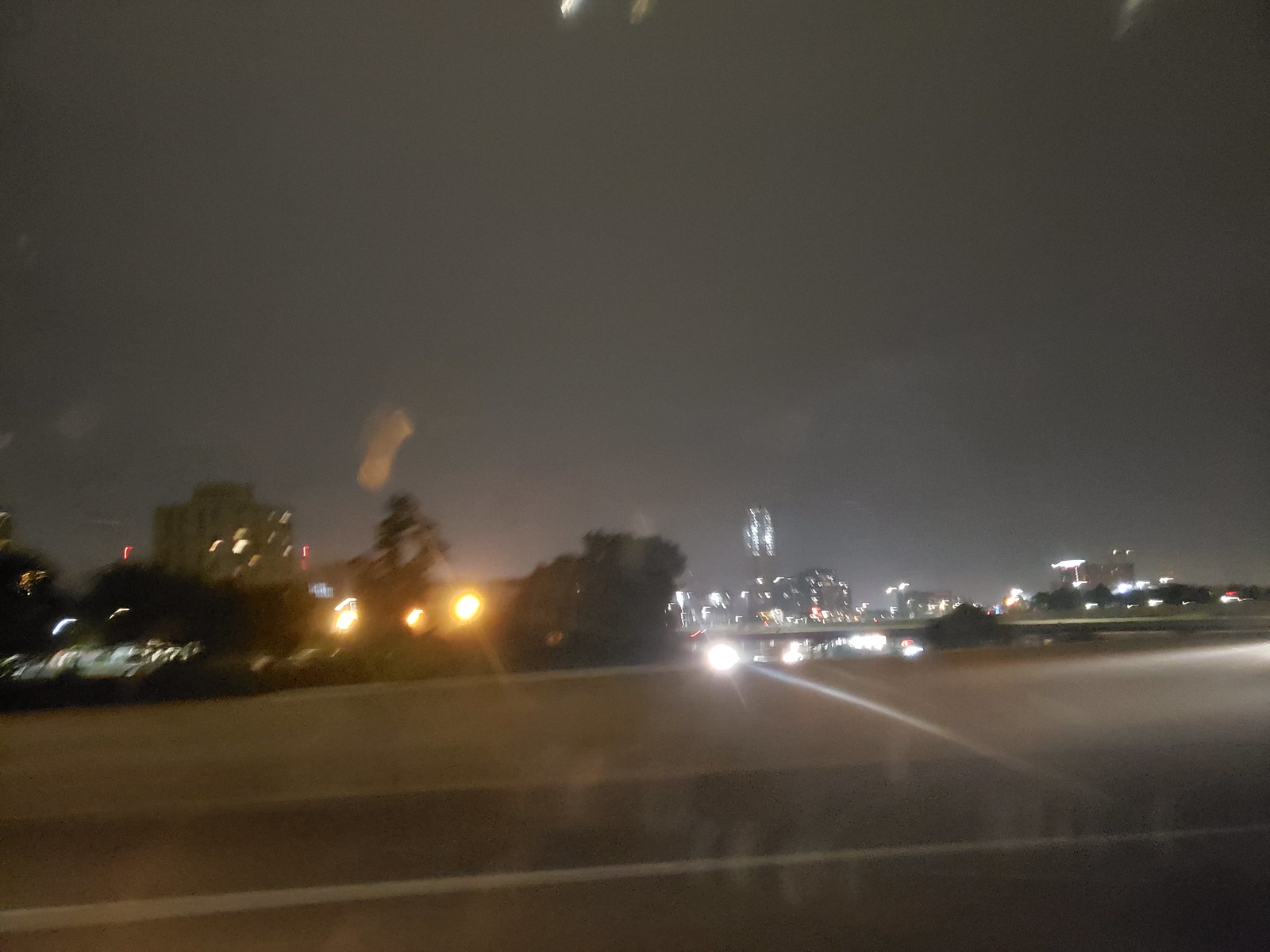The nighttime photo captures a hazy city skyline illuminated by light pollution, with buildings jutting into the dark, cloudy sky, their windows and rooftops glowing. In the foreground, a wide, flat, and empty parking lot is visible, marked by white lines and lit by lights on its right side. Further back, the scene features a bridge with a car driving underneath, headlights glaring towards the camera, and an orange-lit tree line to the left. The image appears slightly underexposed, with some lights blurred from motion, adding a sense of movement likely accentuated by the reflection of glass, suggesting the photo was taken from inside a vehicle.